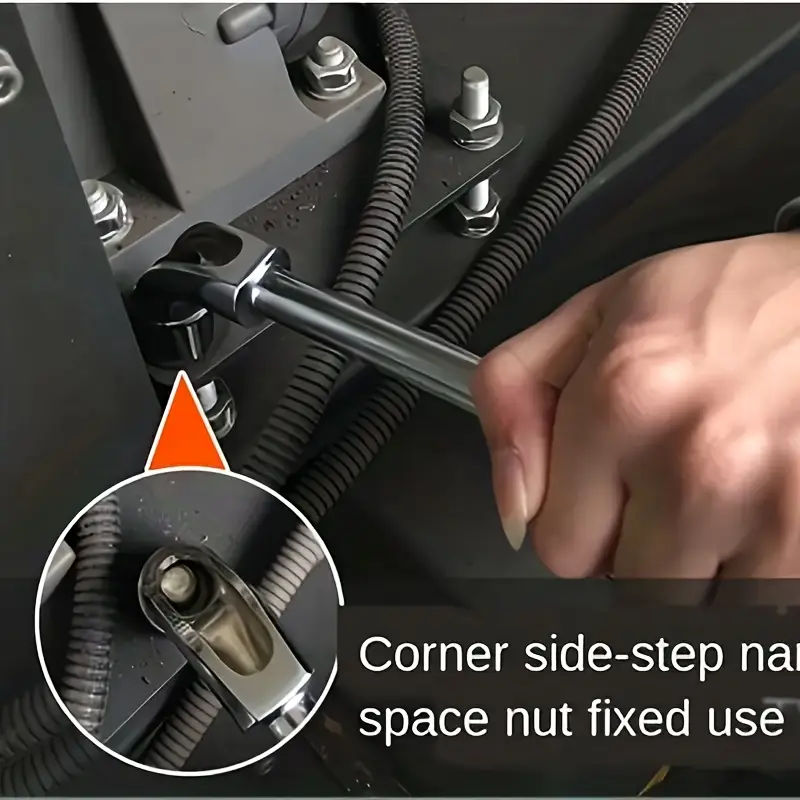This detailed photograph captures a woman's hand, identifiable by her long nails and light skin tone, using a fitted wrench to tighten a bolt on a gray metal assembly. The equipment she's working on includes several nuts, bolts, and a black corrugated hose attached to it, suggesting a piece of machinery that might require regular maintenance. A red arrow in the image points directly to the bolt being tightened, highlighting the focus of her task. The visual is complemented by a close-up inset of the tool engaging with the bolt. Notably, in the bottom right corner, partial text reads "corner sidestep NA something" and "space nut fixed use," perhaps instructions or labels in a manual, reinforcing the technical nature of the scene.